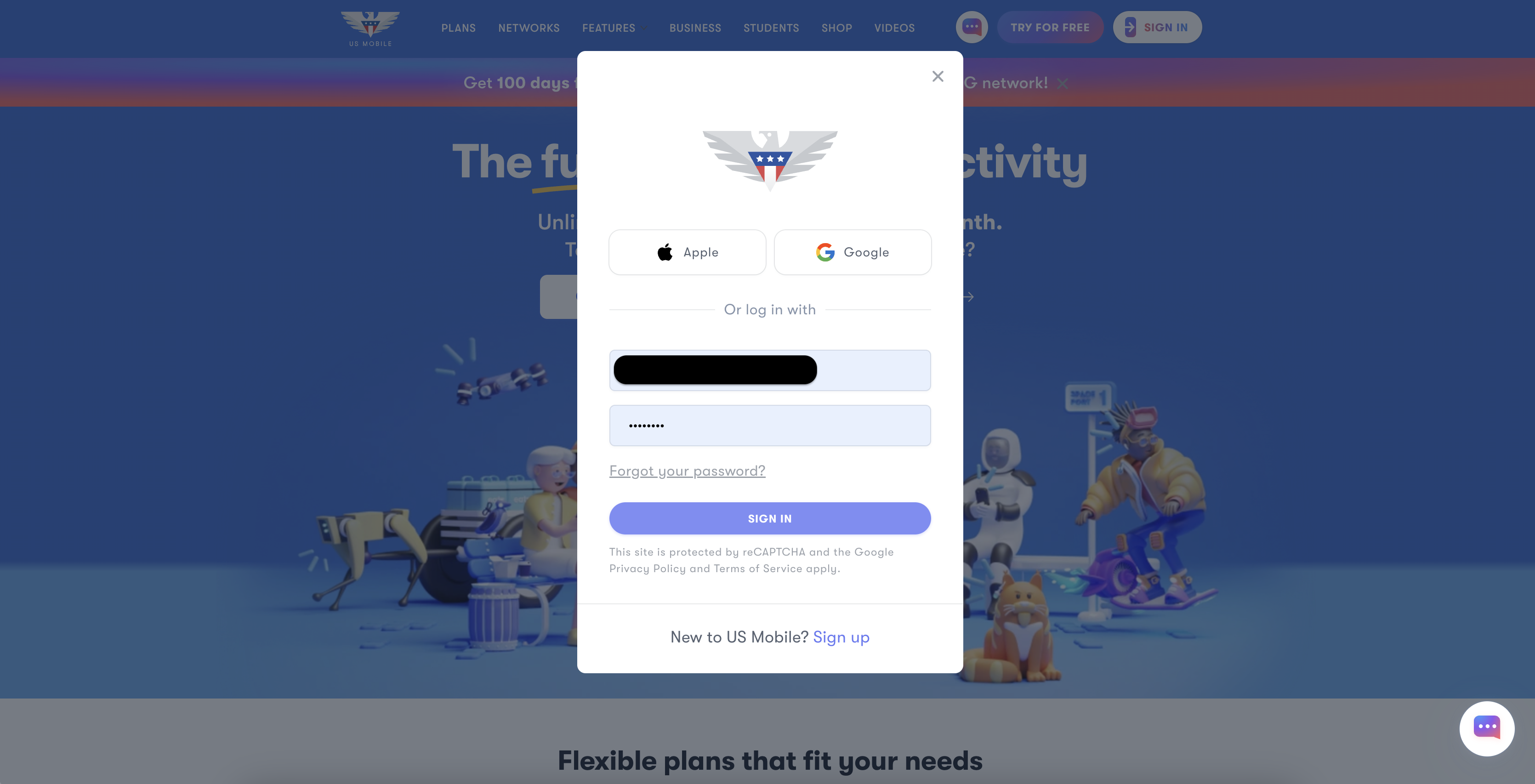The image features a prominent vertical pop-up with a white background, situated centrally. At the top of this pop-up, there's a silver eagle emblematic centerpiece, adorned with an inverted triangle filled with the American flag's red, white, and blue colors, including white stars. Below this emblem, the pop-up displays two horizontal boxes. The left box reads "Apple" accompanied by the Apple logo, while the right box states "Google" next to the Google logo.

Proceeding further down the pop-up, the text "or login with" is visible, followed by two text input fields for entering an email and a password. Beneath these fields, there's a clickable text link that reads "Forgot your password?" with an underline. Adjacent to this link is a button labeled "Sign in." At the very bottom of the pop-up, a prompt encourages new users to sign up, stating, "New to US Mobile? Sign up," with "Sign up" highlighted in blue text.

The background of the overall image is subdued with a blue tint, creating a contrast that emphasizes the white pop-up. Near the upper left corner of the image, the same eagle logo is visible, followed by a series of categories stretching to the right: Plans, Networks, Features, Business, Students, Shop, Videos, Try for Free, and Sign In.